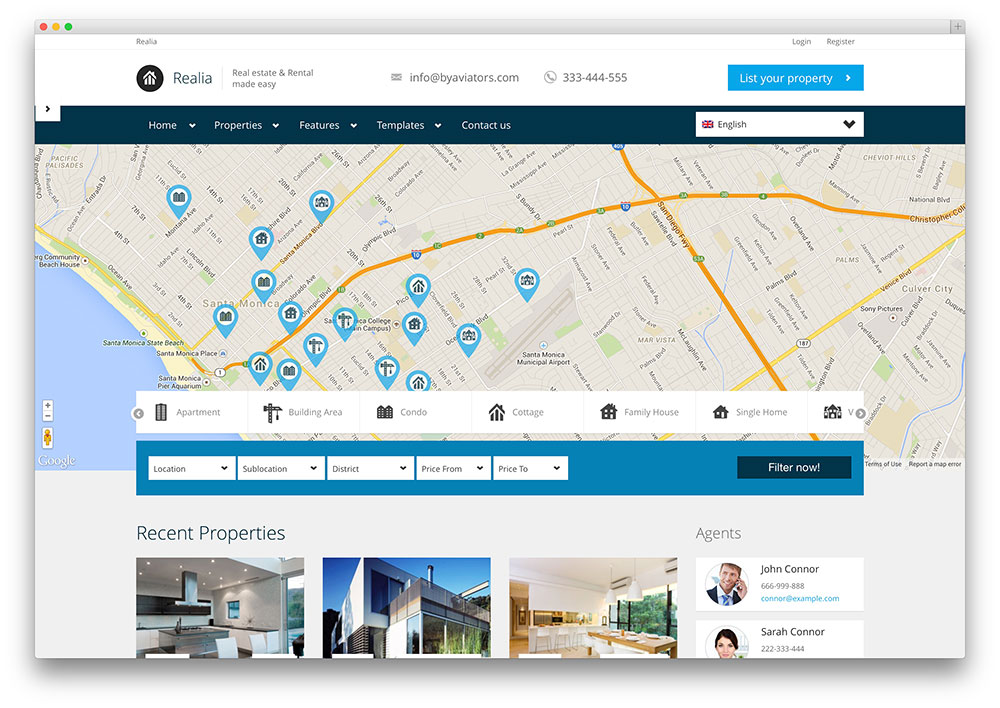Here is the cleaned-up and detailed caption for the image:

---

This is a detailed view of a web page from the website "Relia," specializing in real estate and rentals. On the left side, there's a home icon. The website "Relia" is spelled R-E-A-L-I-A, and their tagline is "Real Estate and Rentals Made Easy." Immediately visible are an email icon with the address info@buyaviators.com and a phone icon with the number 333-444-5555. A prominent blue button labeled "List Your Property" stands out. At the top of the page, there are options to "Login" and "Register."

In the upper left corner, a set of red, yellow, and green buttons is displayed, followed by main navigation tabs under a greenish banner. These tabs include "Home" with a down arrow, "Properties" with a down-facing arrow, "Features" with a down-facing arrow, "Templates," and "Contact Us." Next to these tabs is an English search box.

Below the main navigation is an embedded Google Map with various location icons. Underneath the map are links to different property types such as "Apartment," "Building Area," "Condo," "Cottage," "Family House," and "Single Home."

The site offers filters for users to input their location, sublocation, district (all with dropdown menus), and specify their price range from and to, allowing for more tailored search results. Following this section are photographs showcasing recent properties featuring beautiful, modern architecture. The agents listed for these properties are John Connor and Sarah Connor, with their phone numbers provided.

---